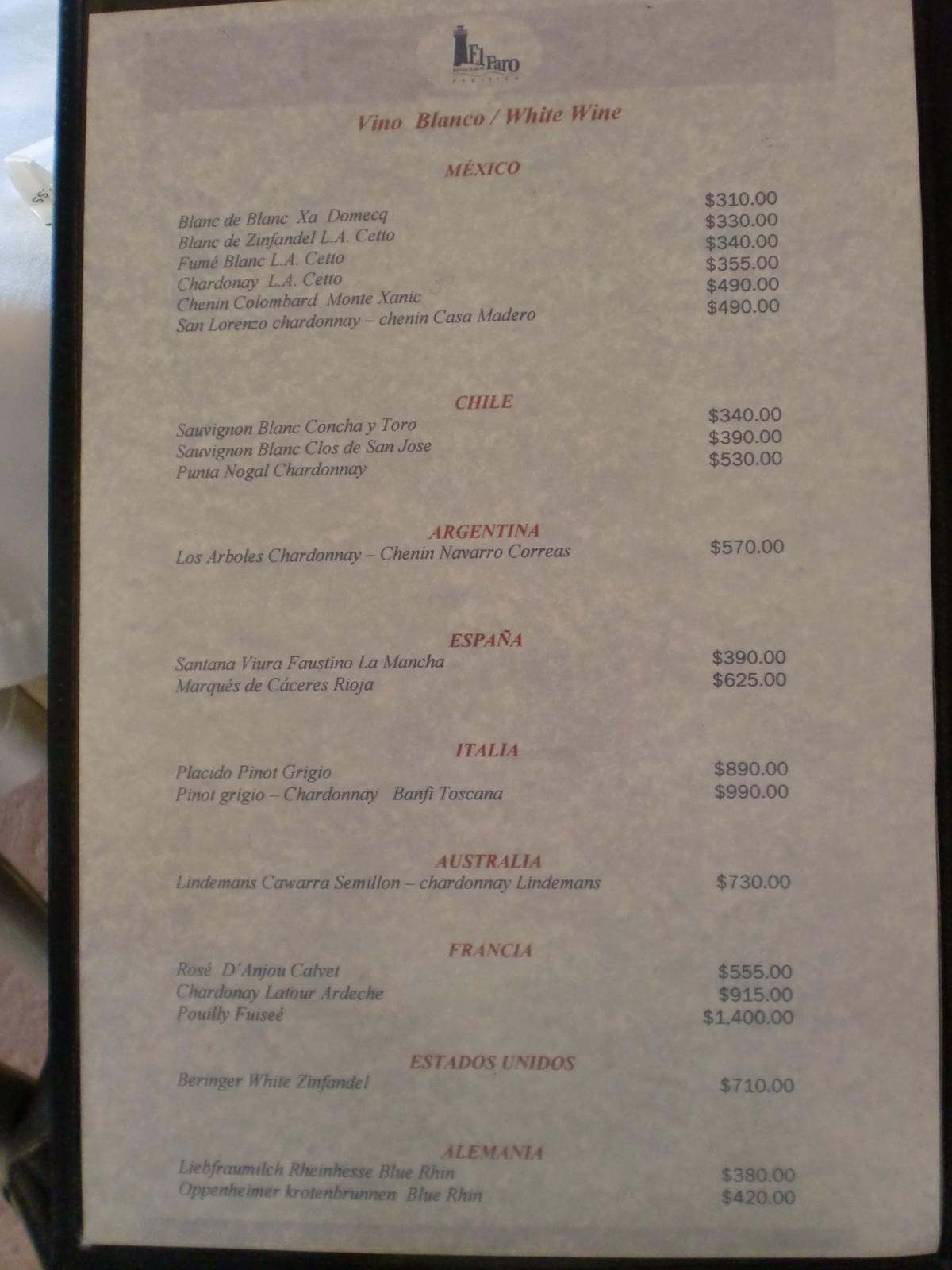This photograph showcases a wine list from El Faro, an upscale restaurant, identifiable by its black logo featuring a lighthouse. The menu is encased in a black-bordered sleeve. The wine selections are categorized by country, with "Vino Blanco" (white wine) prominently displayed in red text. The price ranges for the wines, listed in US dollars, are as follows:

- **Mexico**: $310 to $490 per bottle
- **Chile**: $340 to $530 per bottle
- **Argentina**: $570 per bottle
- **España (Spain)**: $330 to $625 per bottle
- **Italia (Italy)**: $890 to $990 per bottle
- **Australia**: $730 per bottle
- **Francia (France)**: $555 to $1,400 per bottle
- **United States**: $710 per bottle
- **Alemania (Germany)**: $380 to $420 per bottle

The detailed wine list highlights the diverse selection and premium pricing, indicative of the restaurant's high-end status.